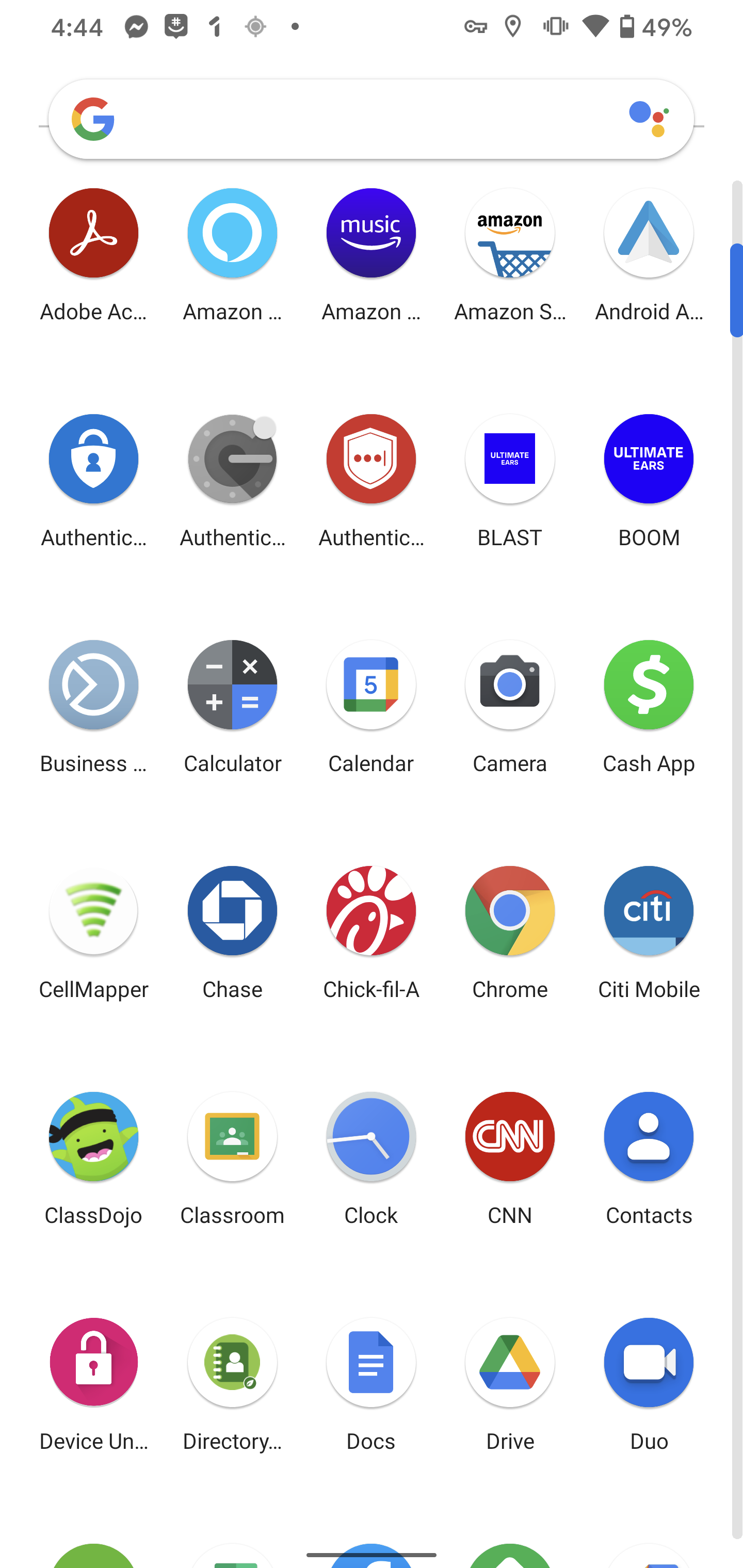This image is a detailed screenshot of a smartphone's home screen, featuring a predominantly white background. A subtle light gray border runs vertically along the right side, starting about an inch from the top and extending to the bottom. At the top of this border, a dark blue strip approximately a quarter of an inch thick captures the eye. 

In the top right corner, the time is displayed as 4:44, adjacent to the icon for a Facebook message represented by a square smiley face with pound signs for eyes. Next to this, a gray circle resembling a scope contains a dot marking 49%, indicating the battery level, which is about halfway full. The Wi-Fi icon shows full signal strength, accompanied by icons for silent mode, location services, and screen lock.

Beneath these status icons is a prominent, rounded search bar branded with the Google logo, which features the familiar color pattern: red at the top, yellow along the side, green at the bottom, and blue traversing upwards and then leftwards. Near the search bar's right edge, several dots in varying sizes and colors are arranged: a large blue dot is followed by a smaller red dot below it, a smaller yellow dot beneath the red, and a smaller green dot above the red.

The main area of the screen is organized into a grid layout, showing five icons across and six icons vertically. Though the detailed specifics of each icon are not fully visible, recognizable icons such as Chrome and Cash App can be identified among them. At the very bottom of the screen, only the top edge of additional icons is visible, hinting at a plethora of apps installed on the device.